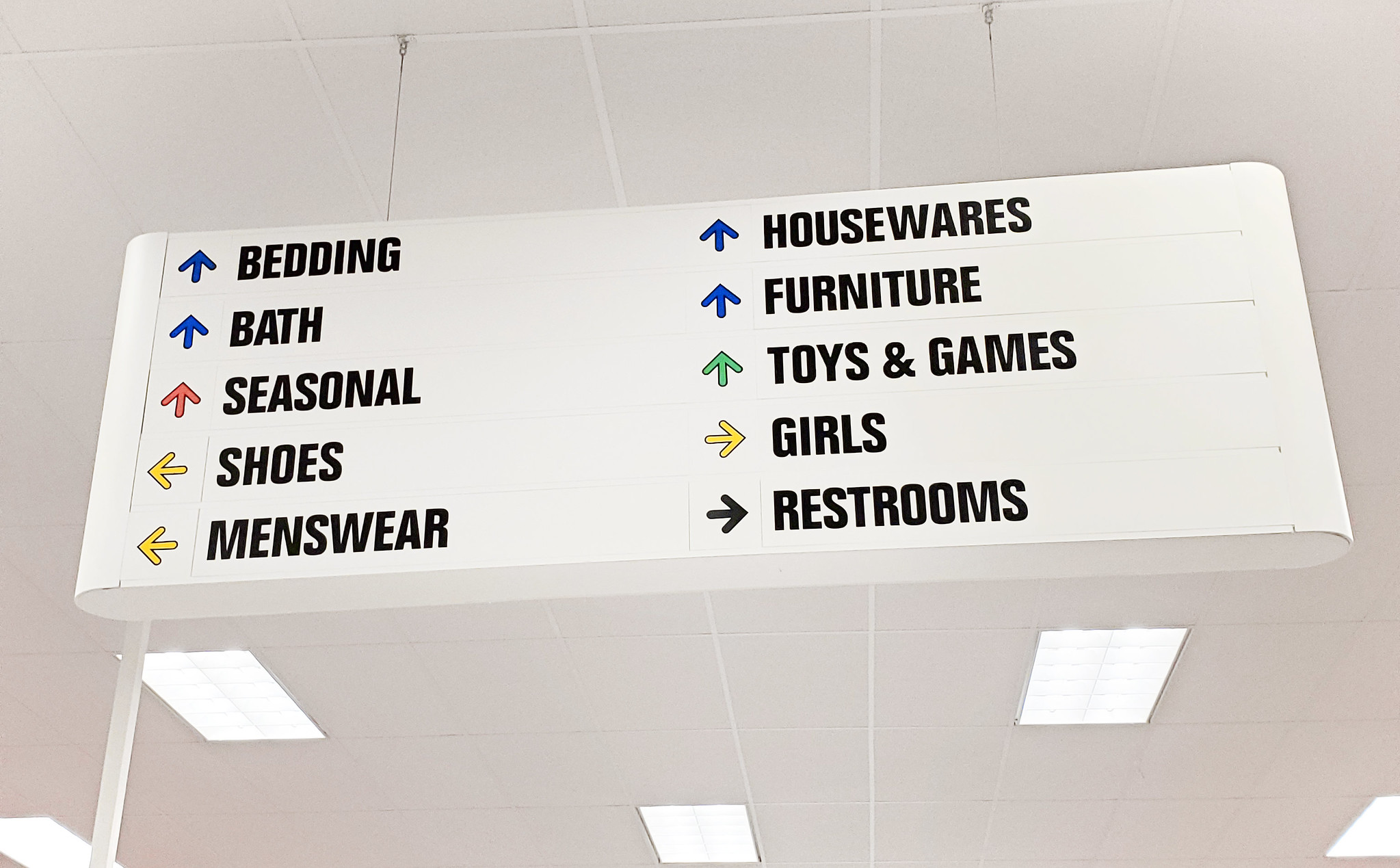A white tile ceiling dominates the top of the image, with evenly spaced light fixtures hanging below it, casting a bright glow over the scene. From the ceiling, a large, pristine white sign descends, featuring multiple directional arrows and clear, concise text to guide shoppers. The top of the sign displays a blue arrow pointing upward, indicating that bedding is located above. Adjacent to it, a red arrow also points upward, directing towards bath items. Nearby, a yellow arrow points to the left, leading to seasonal items, while another yellow arrow points left towards shoes and menswear. To the top right of the sign, several text directives are visible: an arrow pointing upwards towards housewares and furniture, and arrows indicating right towards toys and games, girls' apparel, and restrooms. The left side of the image features a sturdy pole, extending vertically from the floor to the ceiling, providing structural support to the overhead sign.